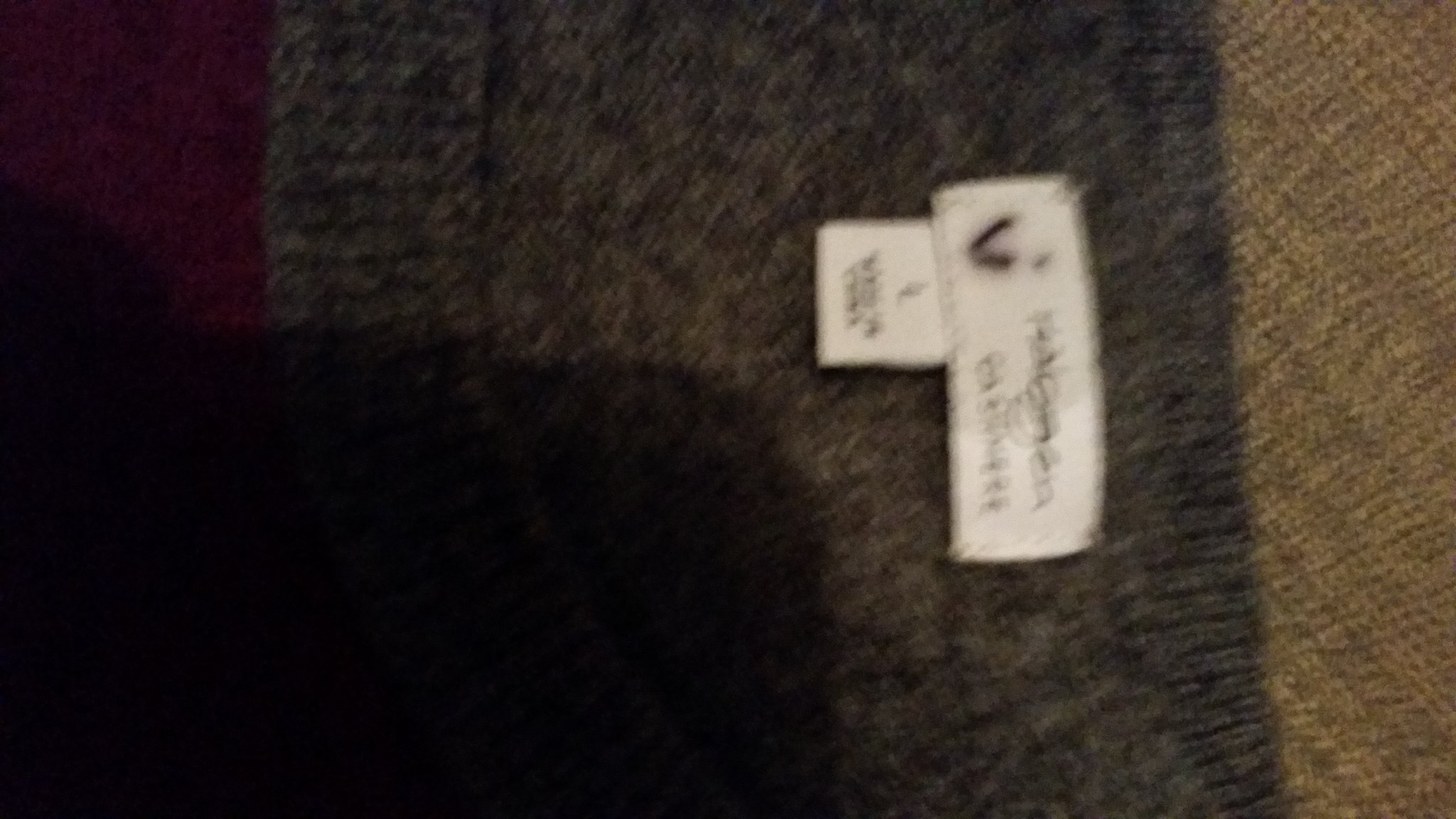This image captures an angled view of a tag on the back of a gray sweater, which is positioned horizontally. The white, rectangular tag is oriented such that the top of the tag points towards the top right corner of the image and the bottom points towards the bottom right. The writing on the tag is out of focus, but a letter "V" can be discerned on the left side. Below this main tag is a smaller square tag displaying a letter "L" followed by some unreadable text in black. The collar of the sweater is also gray, matching the visible back portion. Towards the bottom left of the sweater, a red-colored fabric can be seen. A significant shadow, likely cast by a smartphone, covers the bottom left corner of the image, adding depth and contrast to the scene.